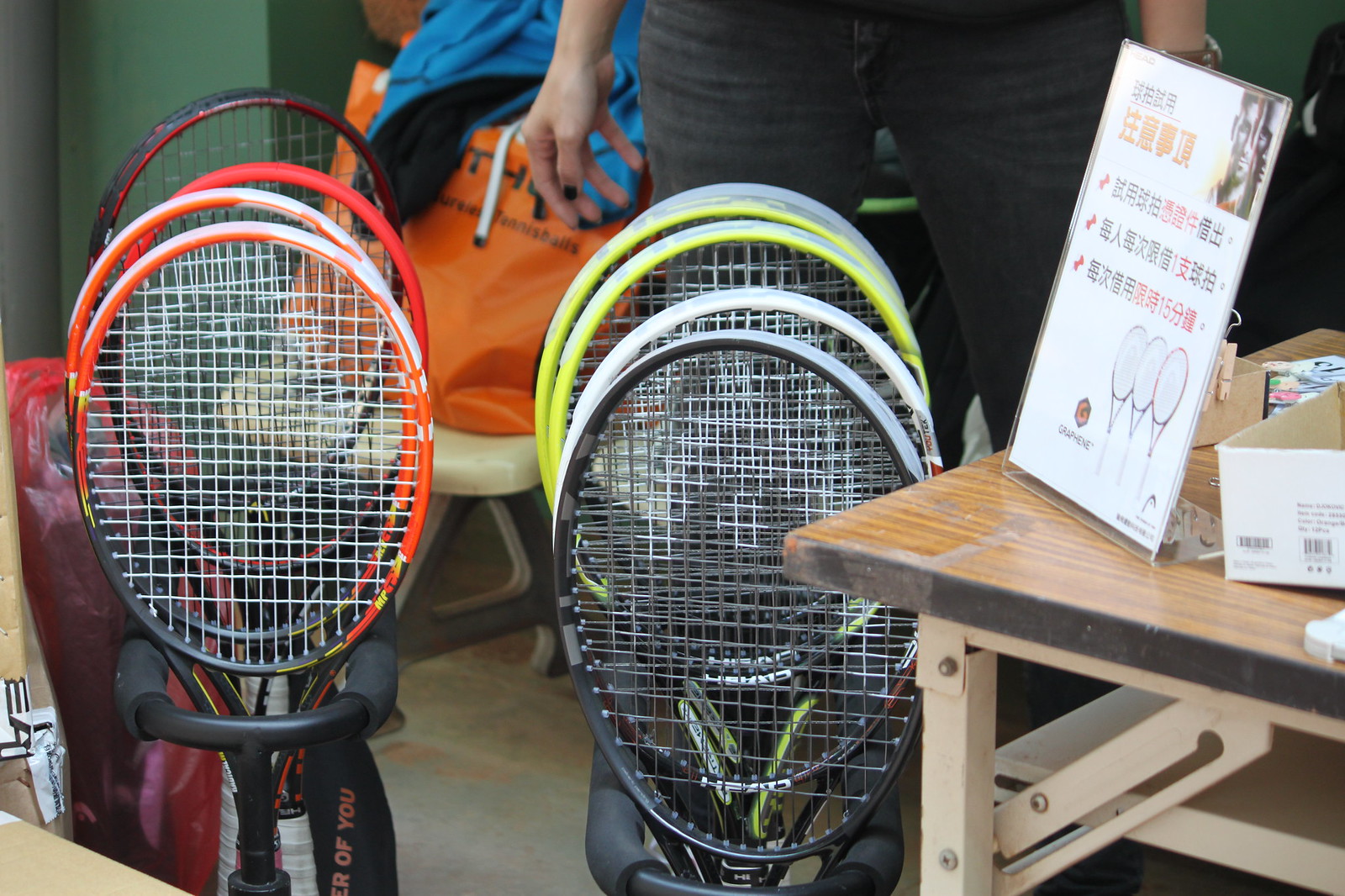This color photograph, taken in landscape orientation, captures an indoor scene centered around several tennis rackets organized in holders. The holders, constructed from black metal piping, display the rackets upright in neat rows. The rackets themselves vary in color, including black-framed ones with tan strings, along with orange, red, yellow, and white variations.

To the right in the foreground, a wooden table with a metal support frame protrudes into the shot. An A4-sized sign in Japanese characters is visible, propped up in a plastic holder on the table, possibly indicating the rackets are for sale or part of a sports lesson display. At the bottom left, three additional rackets lie apart from the others.

In the background, a person, identifiable only from their thighs downward, is standing behind the rackets. They are wearing dark black jeans with horizontal ruffles, and their right hand with painted fingernails suggests they are female. Further back, foldout chairs hold personal items, including an orange bag and a blue jacket, enhancing the sense of a sport center or equipment display area.